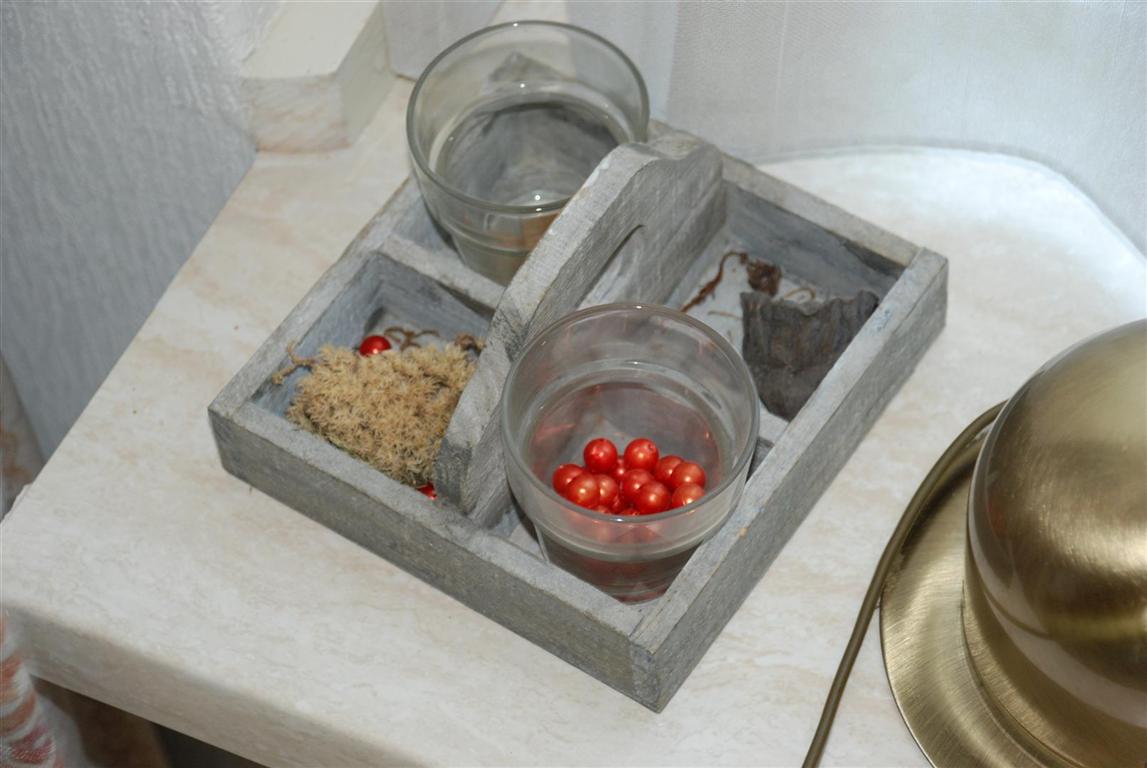This photograph captures a rustic white wooden nightstand with a slightly faded paint finish, revealing hints of underlying brown. The nightstand features a top with a subtle wave design, while the rest of it is straight-edged. The textured white painted wall in the background adds depth to the scene. Resting on the nightstand is a four-section gray wooden carrying tray with a central handle. In the tray’s upper left section, there is a glass of water, while the bottom right section holds a glass containing small red berries. The bottom left section appears to have a mix of berries and a brown, grassy-textured element. The upper right section contains a dark-colored cloth, possibly black or gray. Additionally, a gold-colored metal lid shaped like a hat is placed to the right of the tray, adding a touch of elegance to the rustic setup.